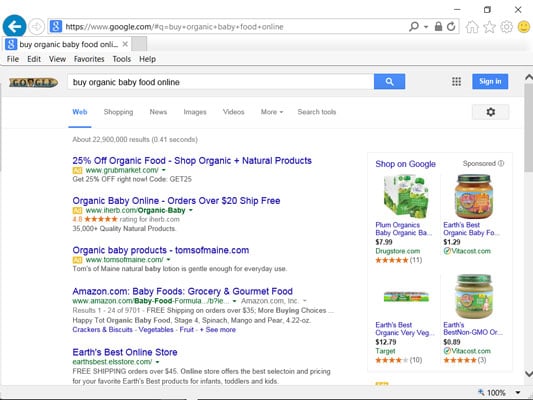A detailed caption for the provided image could be:

"The image displays a web search results page with 'buy organic baby food online' typed into the search bar. The interface offers several navigation options including 'Web,' 'Shopping,' 'News,' 'Images,' 'Videos,' and 'More,' with 'Web' being highlighted in blue. The search results list multiple brands and vendors of organic baby food. The first result from thegrubmarket.com advertises a 25% discount on organic food with the promo code 'get25.' The second link, from Organic Baby Online, offers free shipping on orders over $20 and boasts a selection of over 36,000 high-quality products, all rated with five stars. The third result, from tomsofmaine.com, features organic baby products. Other noteworthy links include baby food options on amazon.com and products from the Earth's Best Online Store. On the right side of the screen, there are images of various baby food products, including two jars of baby food prominently displayed."